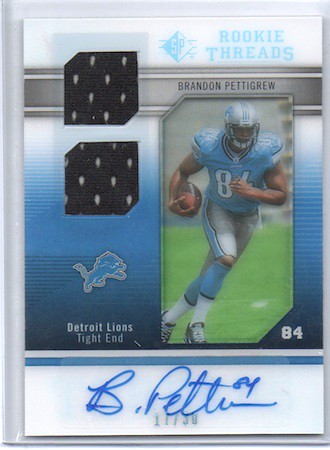This is a detailed vertical rectangular image of a pro sports football card featuring rookie tight end Brandon Pettigrew from the Detroit Lions. The card has a white border, and at the top in large blue letters, it says "Rookie Threads." Adjacent to this, on the right, is a diamond-shaped logo labeled "SP." Below the header, centered, is a photograph of Brandon Pettigrew running with a football, wearing a light blue and silver uniform with the number 84 on his jersey. To the left of the photograph, there are two black dice positioned at various angles, revealing the numbers 8 and 4 with their white dots. Underneath the dice, there is a lion symbol, indicating the Detroit Lions, and it is stated "Detroit Lions, Tight End" in white text. At the bottom of the card, prominently displayed, is Brandon Pettigrew’s signature in blue ink along with his jersey number 84.